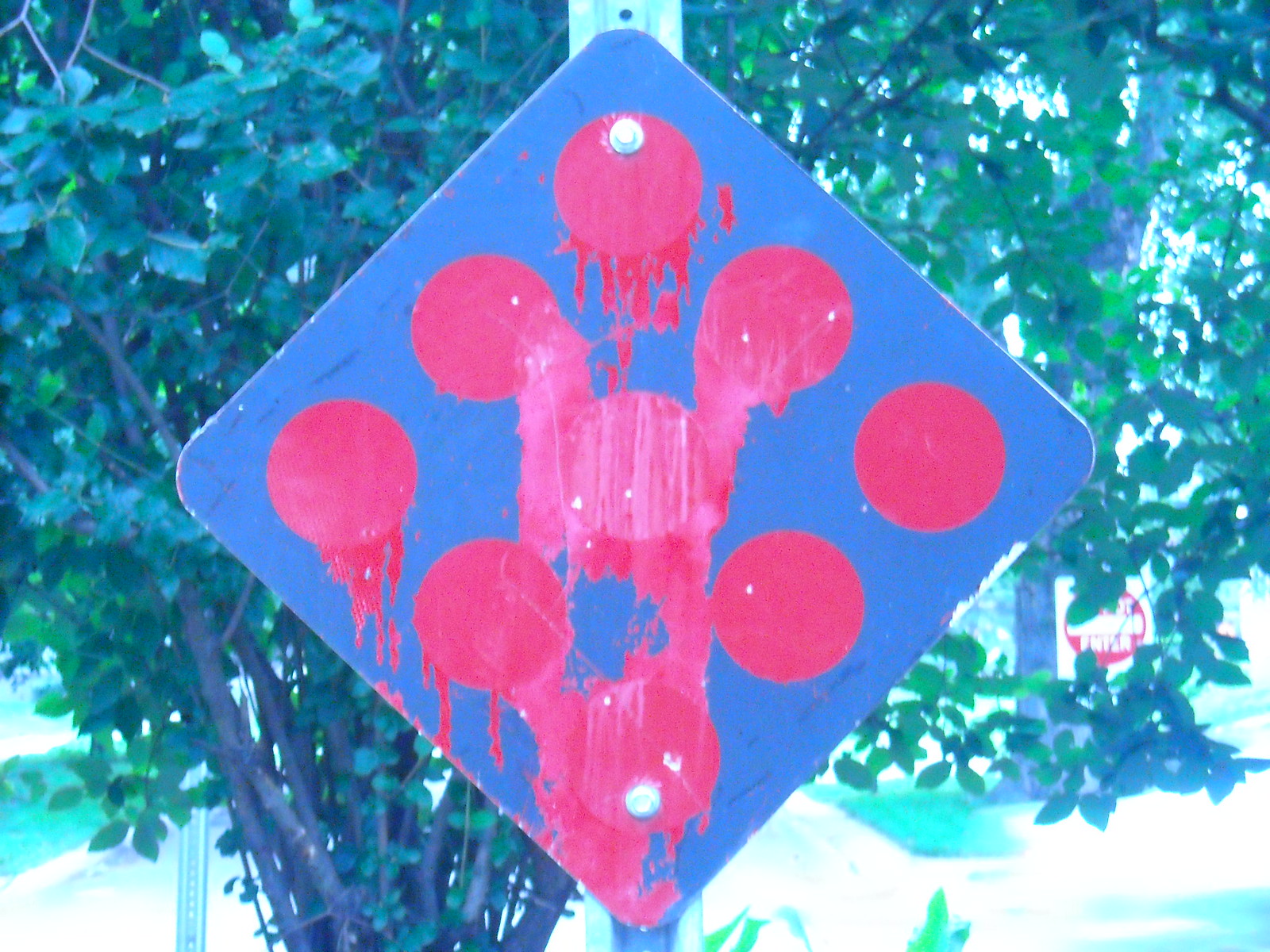This photograph, taken outdoors, captures a detailed and vibrant scene dominated by nature and a distinctive piece of urban art. The background is filled with a dense array of trees that frame both the left and right sides of the image, their dark green leaves providing a lush backdrop. On the right side, sunlight filters through the foliage, illuminating a sign for a store marked by a black outline and a red circle with white lettering.

In the foreground, there is a prominent blue diamond-shaped sign mounted on a metal stand. This sign features nine pinkish-red circles arranged in a diamond formation, each circle distinctively exhibiting streaks of dripping paint, giving them a melting appearance. Notably, the bottom circle is heavily covered with additional red paint. Below this artistic sign, the edge of a sidewalk or road is visible at the bottom of the image. Adding to the urban setting, a "do not enter" red circle sign is partially visible through the leaves on the right side of the photograph. The overall composition creates a striking contrast between the natural surroundings and the intriguing urban artwork.